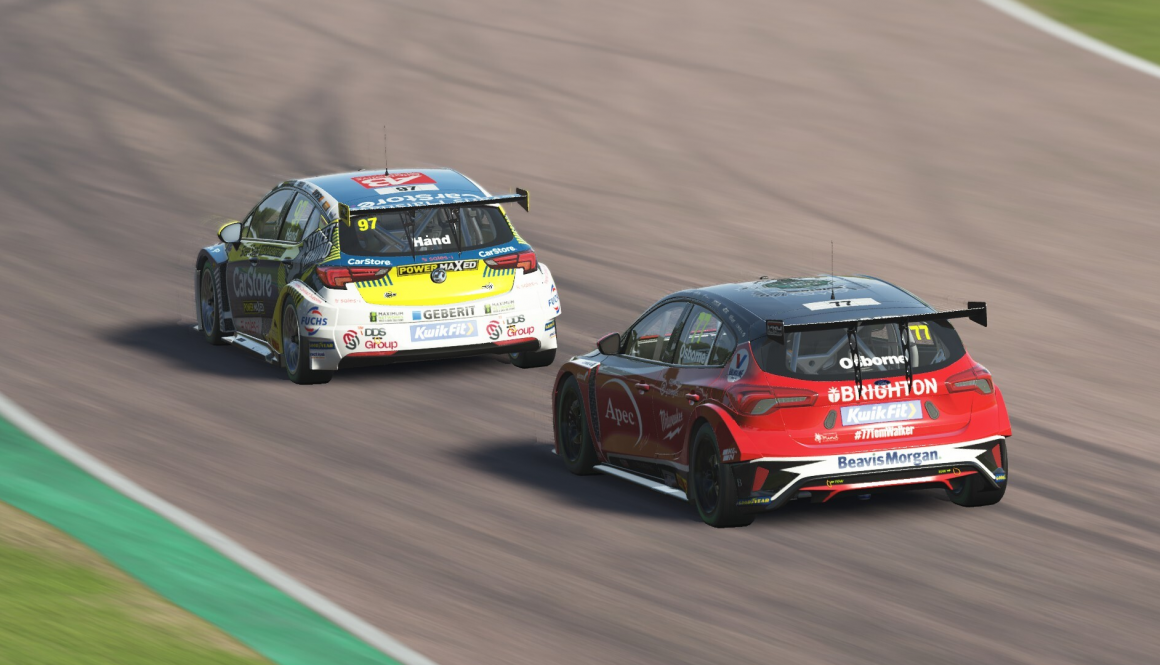This image captures an exhilarating moment on a European racetrack with two colorful, sponsor-laden race cars speeding away from the viewer's perspective. The sleek, black asphalt of the track is marked with tire tracks and shadows, and is bordered by fine white lines and grass-lined strips on both sides, adding a touch of green to the scene. The car furthest to the left is predominantly white with blue and yellow accents, featuring a blue roof, a rear spoiler, and advertisements for companies such as "Gerberit" and "Quick Fit" on the bumper, and "car store" on the driver's side door. Following closely, the car on the right is strikingly red with a black roof and fin. It boasts several sponsorships, including "Brighton" in white letters just below the windshield and across the back, as well as "Epic" on the driver's side door and "Beavis Morgan" on the bottom bumper. Both cars exhibit European license plates, reinforcing the notion that this high-speed duet is occurring on a European circuit.